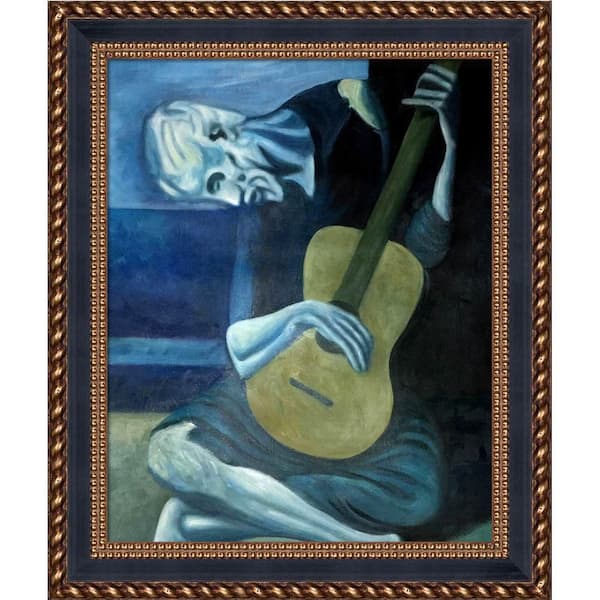This detailed painting, encased in an ornate frame, showcases a spectral figure playing a guitar. The frame features a textured gold outer border, an inner band of dark gray, and a middle layer of beaded gold. The central image reveals an emaciated man with light blue skin and white hair, seated cross-legged on a brown textured surface. He appears ghostly, with white streaks on his skin and hints of hair on his exposed lower leg. His body is bent dramatically forward, almost parallel to the ground, as he plays a yellowish-brown guitar. One hand holds the neck of the guitar while the other mutes the strings. He is clothed in a dark shirt and dark green, olive-hued pants. The background transitions from light to dark blue, emphasizing the man's ghostly presence within the scene.